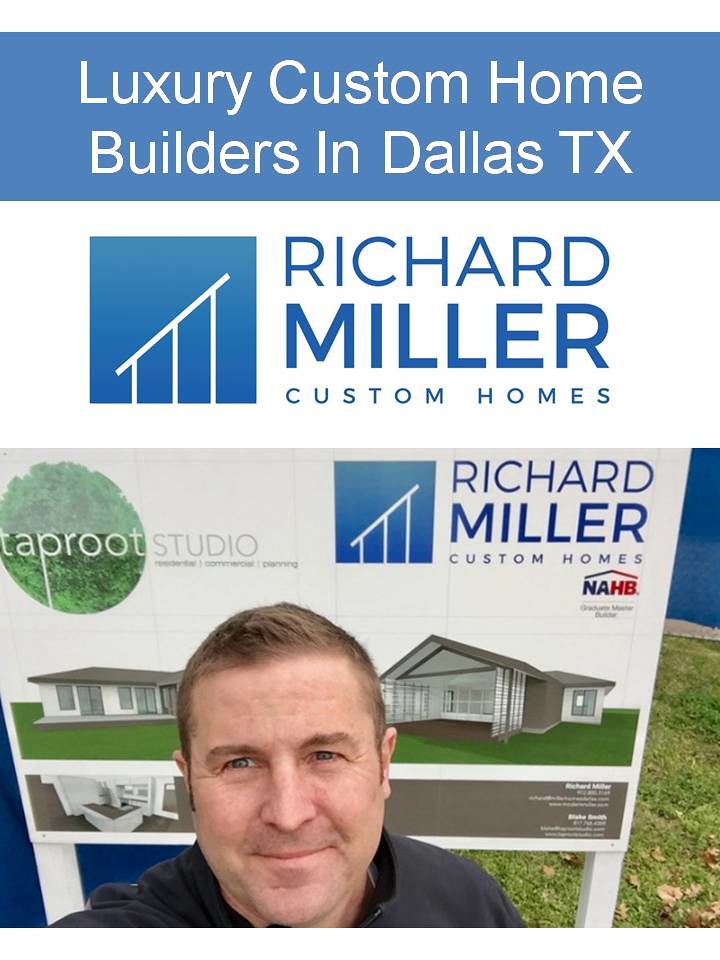This image showcases a man taking a selfie, smiling and looking directly at the camera, while standing in front of a prominent real estate sign positioned outdoors on a grassy area. The backdrop features a large sign with various sections of text. At the very top in a blue strip, white text reads, "Luxury Custom Home Builders in Dallas, Texas." Directly below this strip is an emblem displaying the text “David Miller Custom Homes” in blue letters on a white background. Adjacent to this sign, slightly off-frame, another segment mentions "Taproot Studios," though the full text isn’t completely visible. The scene also includes visuals of newly built homes on the poster, reinforcing the real estate theme. The entire setting, bathed in natural daylight, provides a clear view of the logos, colors (mainly blue, white, green, and tan), and the man who is evidently promoting his real estate business.